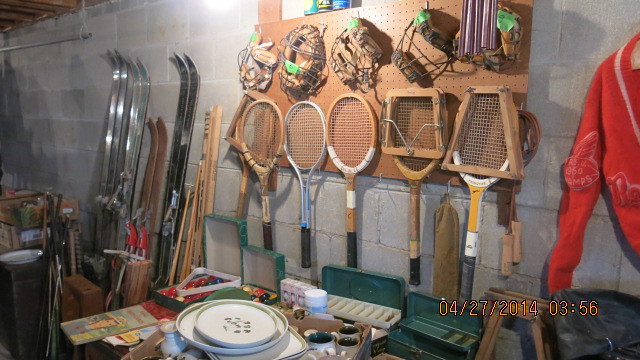The image depicts a cluttered storage area, likely a basement or garage, with a gray cinderblock wall as the backdrop. Central to the scene is a brown pegboard adorned with various sporting goods, including five tennis rackets of different shapes and materials, such as wood and composite, and four metal catcher's masks. To the right, a red sports jacket hangs, partially visible. Below the pegboard, an array of items clutter a table: multiple green tackle boxes, a set of pool balls in a triangular frame within a green case, a book, white plates, and mug settings. On the left side of the pegboard, five sets of skis in diverse colors—black, silver, and brown—lean against the wall. Additional unspecified sports equipment, boxes, and other miscellaneous items are scattered throughout the scene, contributing to the overall sense of disarray. This setting could be interpreted as part of an equipment storage, a garage sale, or an estate sale, with green price tags seen on various items.